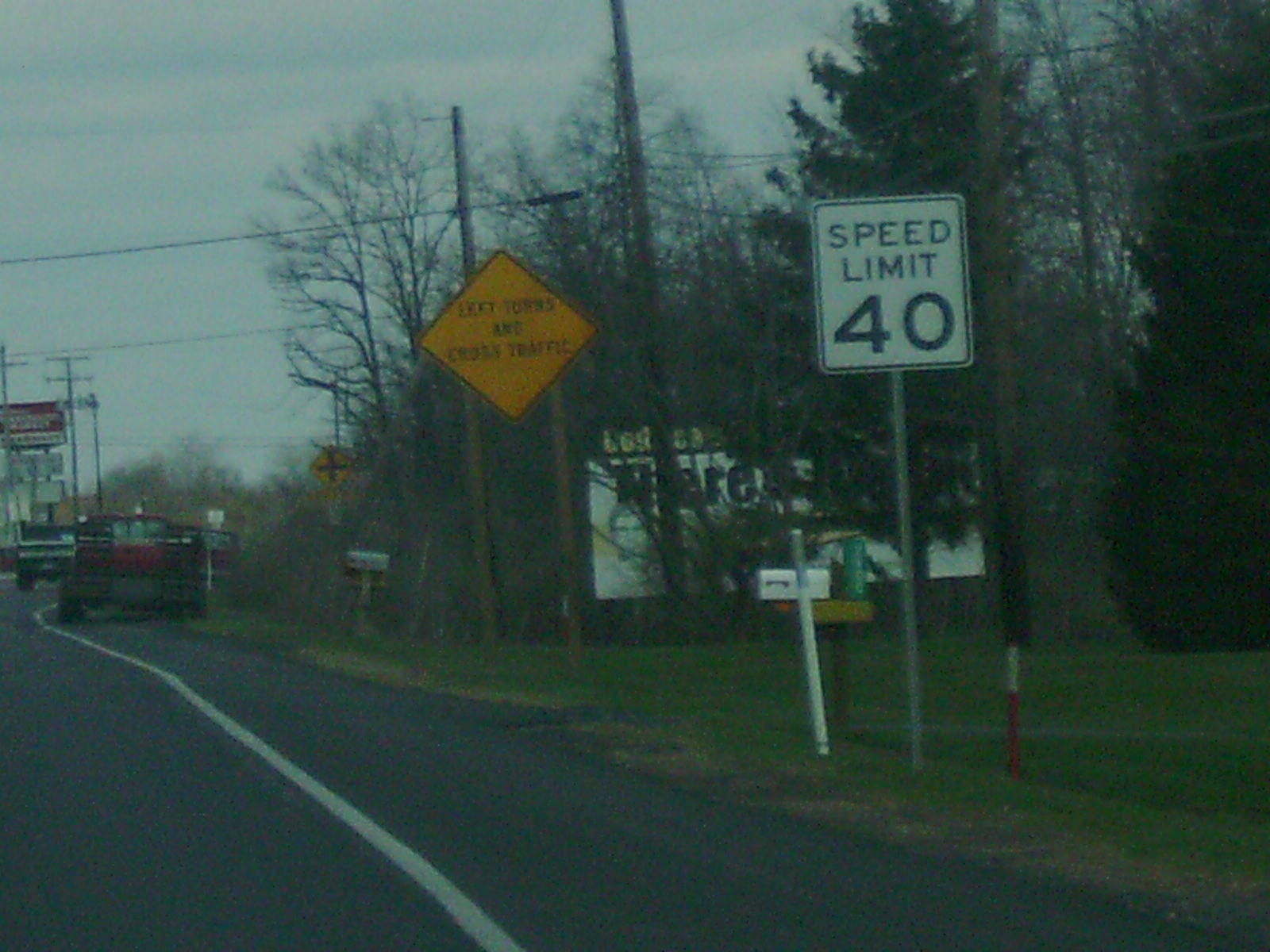In this grainy, dusk-lit photograph of a small town road, the diminishing light casts a muted ambiance over the scene. The composition captures the right lane and its adjacent shoulder, demarcated by a white line. To the right, a flat expanse of grass leads up to a collection of street signs and the silhouettes of trees, beyond which a low-set billboard emerges. 

The first street sign, a rectangular white board with a black border, prominently displays "Speed Limit 40" in stark black lettering. Above it, a gold triangular sign with a black border cautions about turning vehicles and cross traffic. The billboard, partially obscured by foliage, features the image of a man’s face and shoulders on the left side, with the bold black word "HERE" emblazoned above him against a white background.

In the mid-ground, a red pickup truck is pulled over onto the shoulder, and further down the road, another pickup truck continues forward. Flanking the left side of the road, tall marquee signs suggest the presence of a shopping plaza, providing a subtle commercial context to the otherwise tranquil scene.